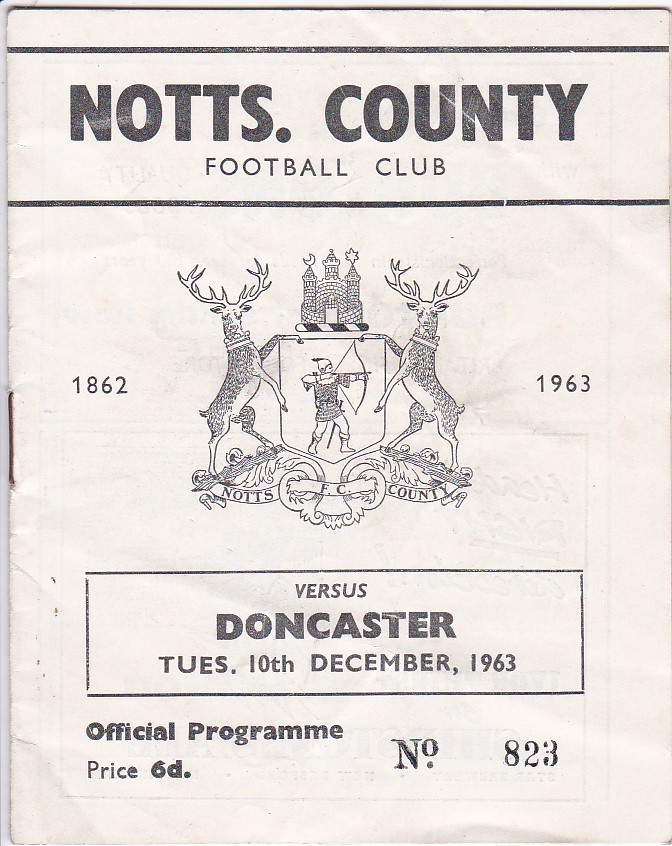The image is a scan of an official soccer program printed on aged, slightly discolored and bent white paper with black text. At the top of the page, the title "N-O-T-T-S County" is prominently displayed, with a smaller, centered subheading reading "Football Club". 

Below the text, a medieval-themed emblem is featured, consisting of a central archer clad in chain mail with a drawn bow, flanked by two deer standing on their hind legs. Above this archer figure, a castle sits with two additional archers, one beneath a moon and the other under a star or sun. 

Additionally, there's a banner at the bottom of the emblem that reads "Knotts FC County." On the left side of the emblem, "1862" is printed, with "1963" to the right. Further down the paper, within another text box, it indicates the match details: "Versus Doncaster, Tuesday, 10th December 1963." The bottom left of the paper states "Official Program, Price 6D," and the bottom right is marked with the number "823."